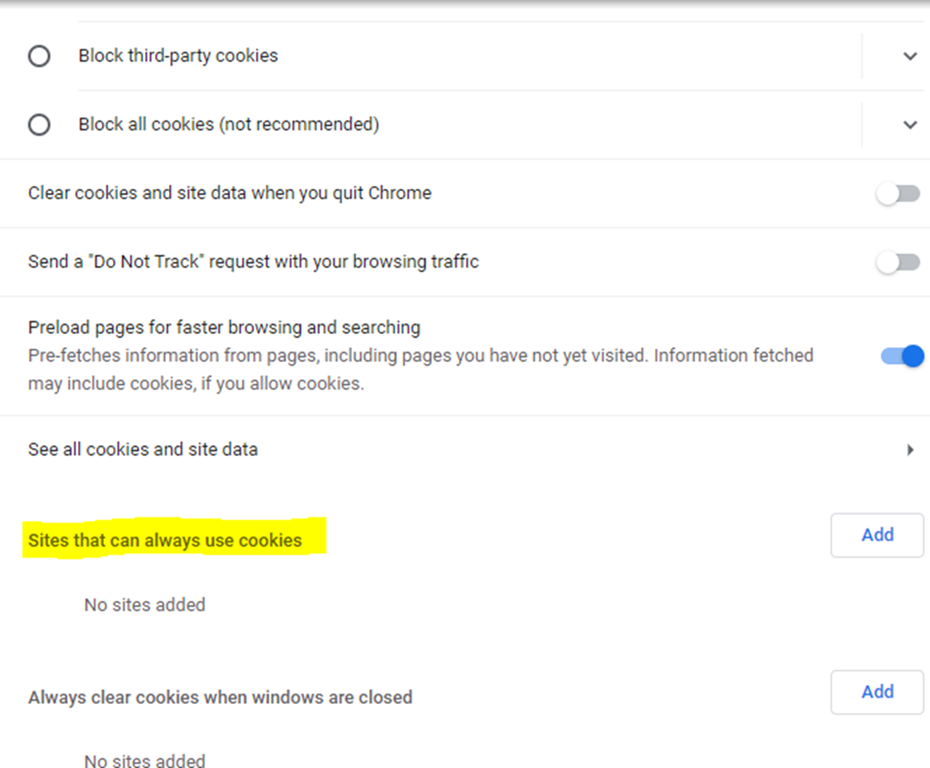The image shows a detailed view of the Privacy and Security settings in Google Chrome. The settings displayed include options to block third-party cookies and the recommendation to avoid blocking all cookies. Users are given the option to clear cookies and site data when they quit Chrome, and can send a "Do Not Track" request with their browsing traffic. Additional features include preloading pages for faster browsing and searching, which involves pre-fetching information from pages not yet visited. If cookies are allowed, this pre-fetched information may include cookies. Users can view all cookies and site data, manage sites that are always permitted to use cookies, and ensure no sites are allowed by default. There is also an option to always clear cookies when the browser windows are closed, with an indication that no sites have been added to exceptions.